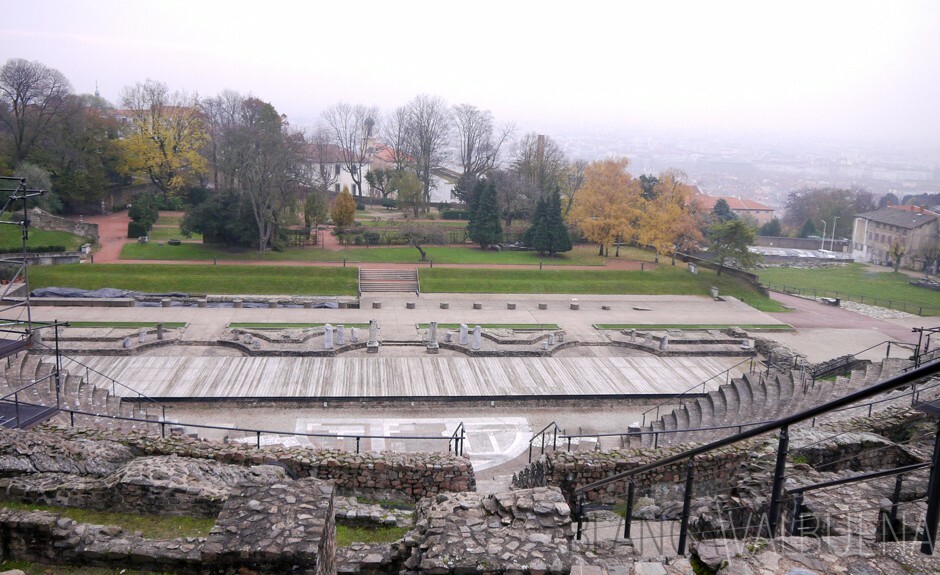The photograph depicts an outdoor amphitheater that appears to be repurposed from ancient ruins. The audience seating area is characterized by worn stone staircases, with modern black metal railings running down the steps. Multiple eroded and broken stone walls frame the scene, contributing to the sense of historical decay. Near the bottom of the amphitheater, there is a flat, marble-covered area leading to a raised modern wooden platform, suggesting a contemporary stage setup. Scattered around the stage are various broken marble pillars, remnants of the structure that once stood there. Further in the background, steps descend to a red brick pedestrian path that is flanked by trees and hints of a wooded area, with some houses and buildings visible through a light fog. The sky is hazy white, adding to the atmosphere of faded grandeur. The overall color palette includes whites, grays, blacks, reds, oranges, and tans, reflecting both the ancient ruins and the modern interventions. This setting maintains an air of tranquility, possibly frequented by joggers or walkers navigating the stone steps amidst the historical remnants.